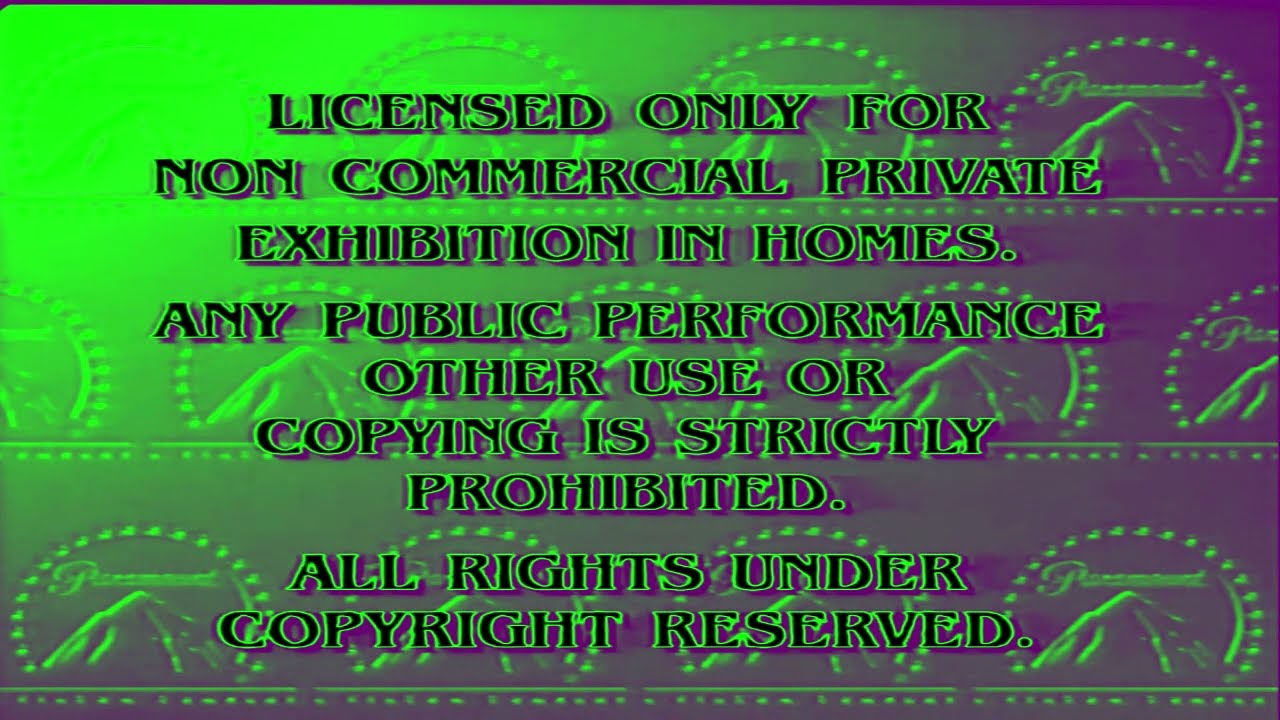This image appears to be a screenshot taken from the beginning of a movie, showing the familiar copyright warning seen in most home-viewed films. The text, written in uppercase black font with green outlines, states: "LICENSED ONLY FOR NON-COMMERCIAL PRIVATE EXHIBITION IN HOMES. ANY PUBLIC PERFORMANCE, OTHER USE, OR COPYING IS STRICTLY PROHIBITED. ALL RIGHTS UNDER COPYRIGHT RESERVED." There are nine lines of text in total. The background features a repetitive pattern of the Paramount Studios logo, with the iconic mountain and stars. This pattern is arranged in three rows: three logos at the top, five in the middle, and four at the bottom. The color scheme is predominantly green in the upper left area and purple in the lower right, with the colors blending diagonally across the image, giving a mixed appearance in some spots. The top row of logos is mostly green, shifting to a mix of green and purple, and finally to purple. The middle row shows a similar transition, with initial logos being green and gradually including more purple, while the bottom row is predominantly purple with some green accents. This vividly colored background creates a dynamic yet familiar scene typical of pre-movie copyright screens on DVDs intended for home use.